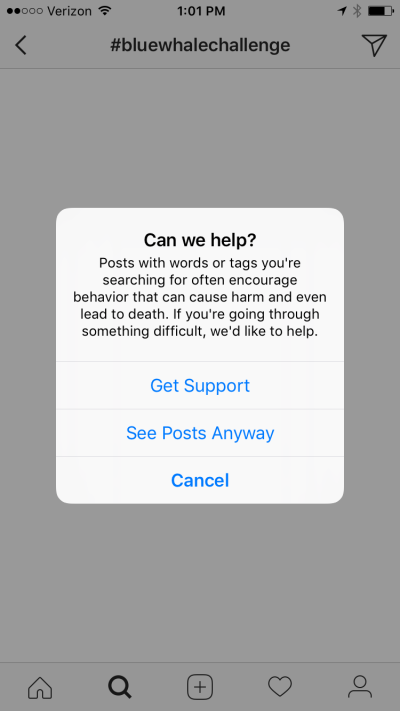The image displays a gray background featuring several interface elements. At the top, there are five dots, two of which are black, indicative of a notification or status bar. Near these dots, the text "Verizon" and the time "1:01 p.m." are prominently displayed. To the right of this is a left-pointing arrow, the hashtag "#BlueWhaleChallenge," and a small airplane icon pointing to the right, signifying a message or navigation feature.

Beneath these elements lies a large white box with a message designed to offer help. The text within the box reads: "Can we help? Posts with words or tags you're searching for often encourage behavior that can cause harm and even lead to death. If you're going through something difficult, we'd like to help." Below this, there are three clickable options delineated by thin lines: "Get Support" in blue text, "See Post Anyway," and "Cancel."

At the bottom of the image, a menu bar displays five icons on the gray background: a house representing the home screen, a magnifying glass for search, a square with a plus sign for adding new content, a heart for likes, and a small person icon for user profile.